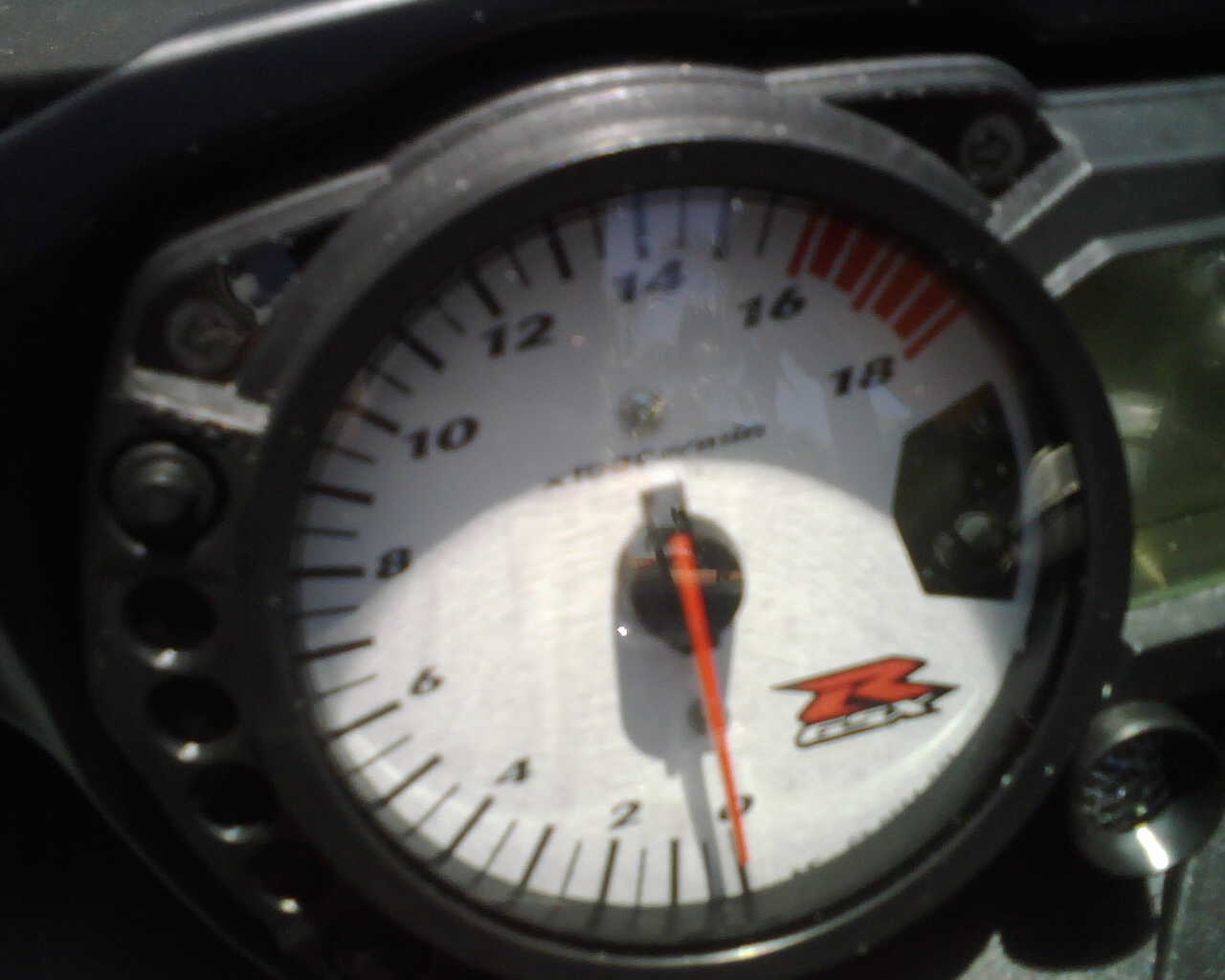A blurred outdoor photograph captures a vehicle's gauge, brightly illuminated by overhead sunlight. The dial, presumed to be a rev counter, is set against a black plastic backdrop. It features white numerals in 2-unit increments from 0 to 10, with a needle poised in red, emanating from a central black circle. The recessed screen of the dial casts a partial shadow over the face, accentuating the depth. The upper right portion of the dial shows markings in red, indicating critical levels between 16 and 18. The bottom right of the dial bears a distinct logo, showcasing a red "R" with additional, indiscernible white text outlined in black, giving it a three-dimensional appearance.